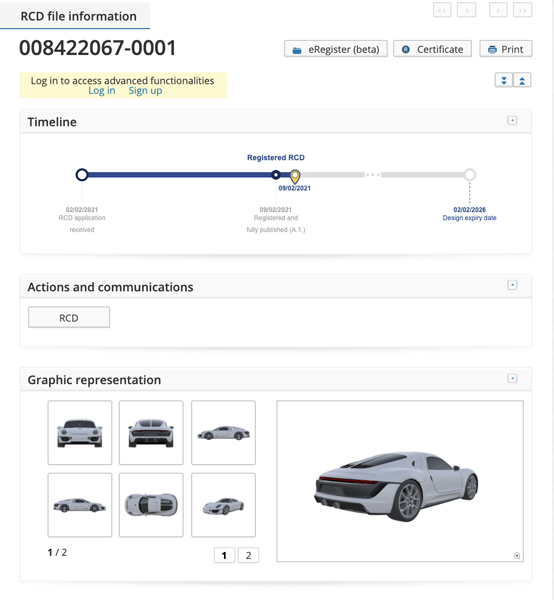The image displays a website interface with a series of functional tabs and buttons designed for user interaction. At the very top, there's a tab titled "CD File Information," indicating the section of the site you are currently viewing. Immediately below this, a unique identifier number "008422067-0001" is prominently displayed. 

To the right, there are three buttons: "Register Beta," "Certificate," and "Print," providing users with various options for document interaction. Beneath these buttons, a prompt reads "Log in to access advanced functionalities," accompanied by log-in and sign-up links for user authentication.

Further down, there's a wide box spanning horizontally across the page, labeled "Timeline," which appears to guide users through a registration process for RCD. The timeline is visualized with three checkpoint circles numbered one, two, and three, indicating steps in a sequence.

Following the timeline section, there's a labeled bar titled "Actions and Communications," serving as a header for subsequent content. Below this header, the image features a photograph of a white car, likely relating to the subject matter of the page.